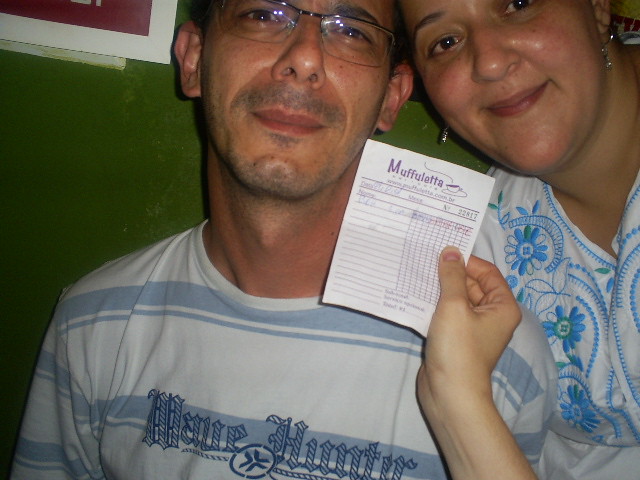This square photograph is a close-up of a man and a woman standing closely together against a green wall, which has a red sign with a thick white border hanging on it. Both individuals are smiling softly with their mouths closed. The man's narrow wire-rimmed glasses are visible, along with one of his eyebrows. He's wearing a blue and white striped shirt that has some text on it, appearing to say "Maui Hunter," though the design makes it hard to read clearly. The woman next to him, who also has her head slightly cropped by the photo, has brown eyes and no glasses, and she is dressed in a white top with a blue floral pattern. One of them is holding up a small rectangular receipt to the camera. The receipt reads "Muffaletta" at the top, accompanied by a small image of a cup and saucer with steam rising from it. The image suggests an indoor setting, probably a restaurant, and is lit in a way that hints at a dim ambiance.